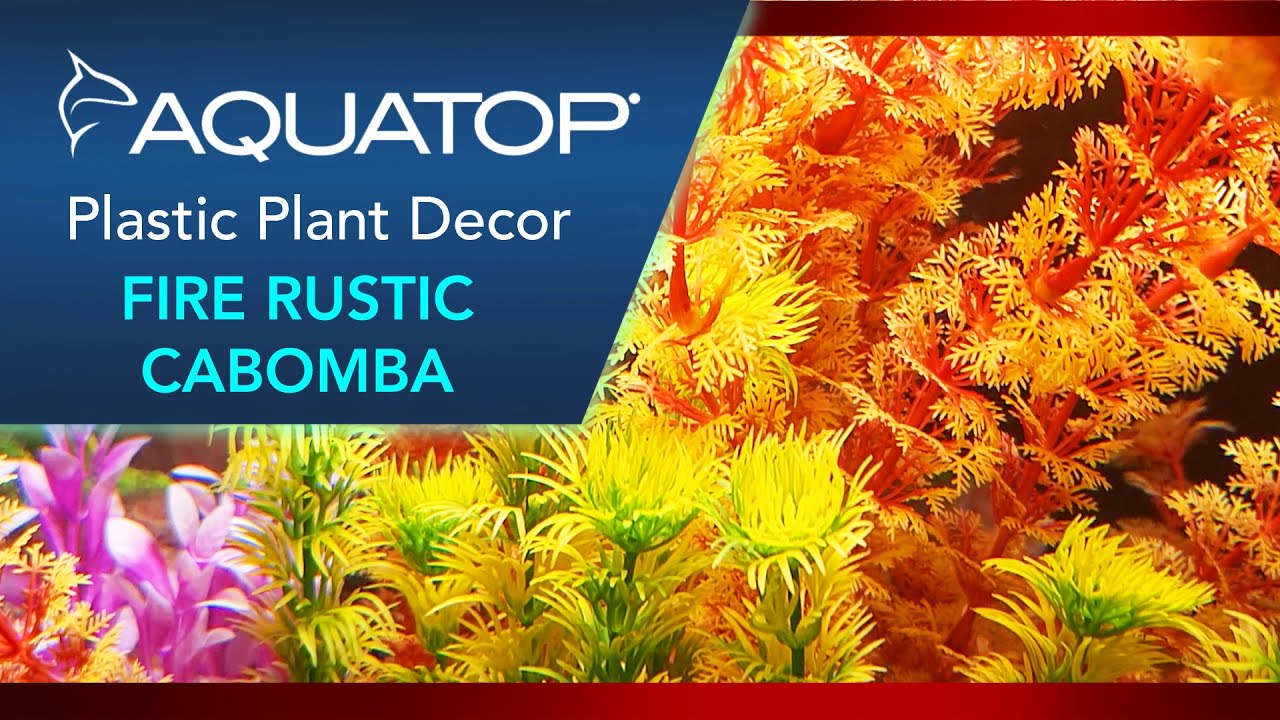The advertisement for Aquatop's Plastic Plant Decor, prominently displayed in a rectangular image, features a blue section in the upper left-hand side with a small drawing of a shark and the text "Aquatop." Below, it reads "Plastic Plant Decor" in white, and then "Fire Rustic" and "Cabamba" in blue lettering. To the right of this blue area, the majority of the picture showcases a lush array of realistic-looking plastic plants. Predominantly, these plants have green stems with vibrant yellow foliage, supplemented by some with red stems and yellow fronds. There are additional splashes of color throughout the scene: blue flowers on the left, violet flowers in the lower left corner, yellow flowers in the lower right and center, red flowers in the center, and orange flowers in the upper right and upper center. The diverse, vivid colors and detailed variety aim to captivate potential purchasers, making it an attractive option for room decor that lasts.